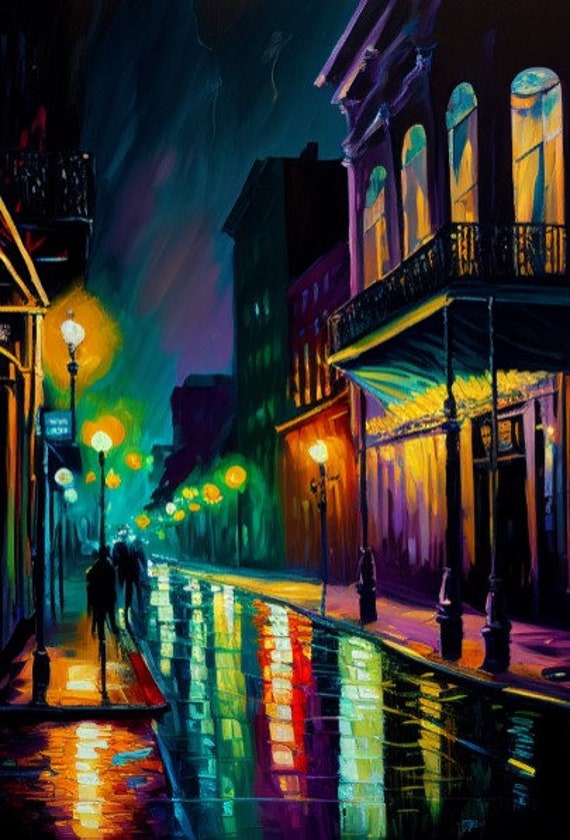The image is an impressionistic painting capturing a vibrant, nighttime city street with a surreal and almost dreamlike quality. The scene is dominated by a dark black sky with hints of purple streaking upwards, adding to the atmosphere of the night. The composition is taller than it is wide, making the vertical elements more pronounced. A road stretches from the front right corner and middle of the picture, narrowing to a point halfway up the painting, creating a strong perspective effect.

Streetlights line both sides of the road, casting radiant light that reflects on the glistening, wet surface of the street. These reflections create a dazzling array of colors—blues, yellows, oranges, green, and pinks—forming a mosaic of hues on the pavement. The sidewalk, also illuminated by the city lights, displays these reflections vividly, enhancing the surreal ambiance. 

On the left side, indistinct figures walk away, adding life to the scene without detracting from the focus on the vibrant surroundings. Buildings on both sides of the street feature balconies with wrought-iron railings and arched windows, evoking a sense of New Orleans flair. The overall effect is a captivating representation of a bustling city night, rich with color and reflection.